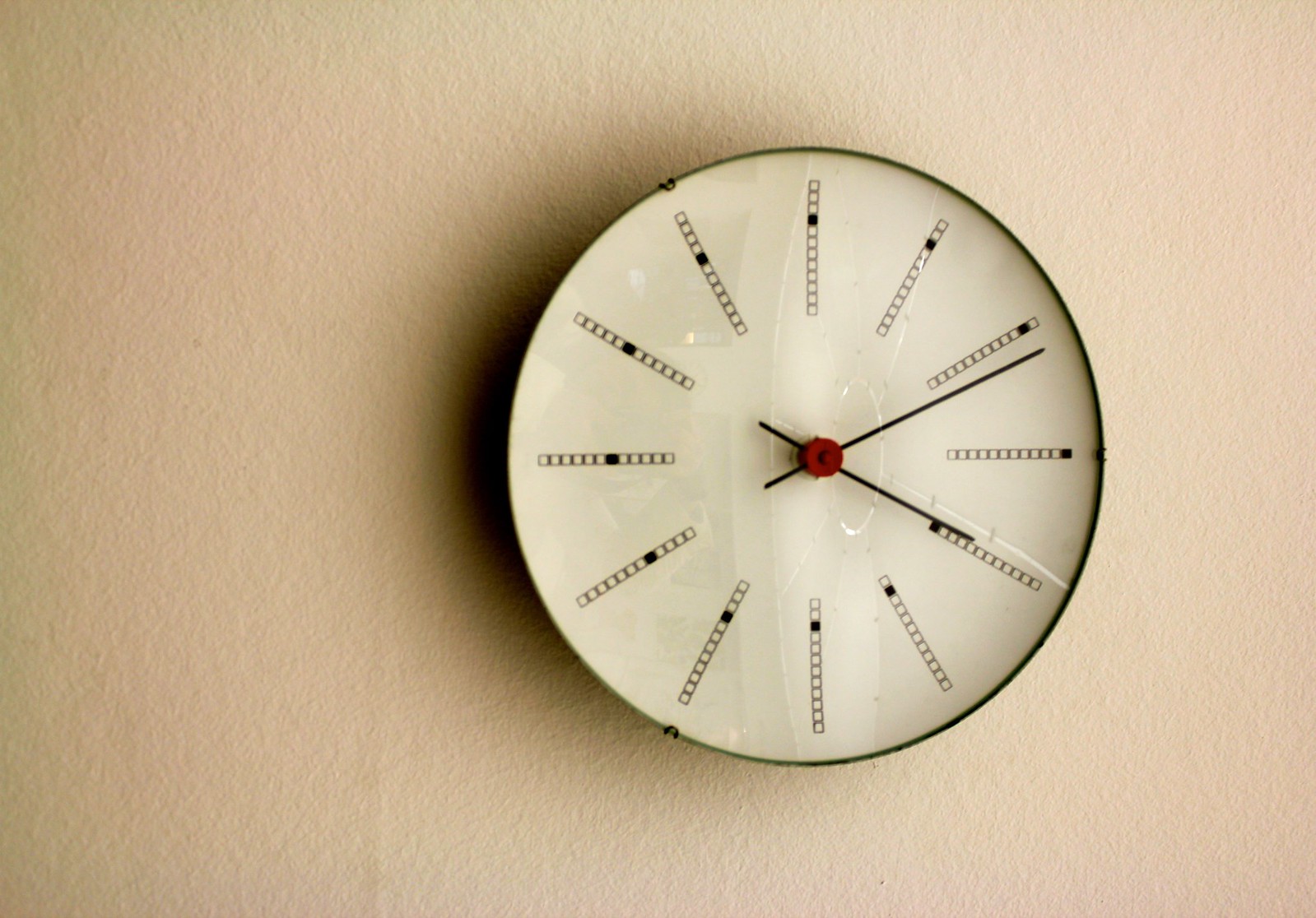This image captures an abstract, analog clock mounted on a beige wall. The clock features a small black circular frame and a white face. The clock face is unique, presenting twelve rectangular black lines that resemble ladders, each with one segment filled in to mark the hours. The lines radiate from a central red circle, contributing to the clock's modern and geometric aesthetic. Showing the time as 4:11, the clock has black minute and hour hands, with no second hand present. The white background of the clock face has a slightly wrinkled texture, and the beige wall casts a shadow to the left, accentuating the clock's three-dimensional effect. A subtle dimple or crease is noticeable on the wall, adding to the image's detailed composition.